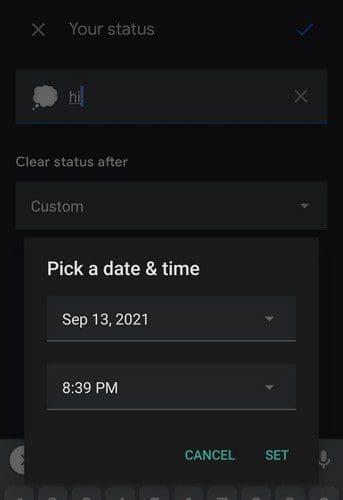The image features a user interface with a predominantly black background. In the upper left corner, there is a gray 'X' icon. To the right of this icon, the words "Your Status" appear in gray text. Further to the right, a faded gray checkmark suggests that this option is likely disabled.

Below this section, a field with a dark gray background contains a thought bubble icon in light gray on the left. Inside the bubble, the user has typed "hi" in lowercase, light gray letters, which are underlined. The cursor is positioned next to the "i," indicating the user is still typing. On the right side of this field, there is a light gray 'X' icon.

Underneath this input field, the background reverts to black. On the left, in small gray text, it reads "Clear status after." This line leads into a dropdown menu with a dark gray background. On the left side of the dropdown, "Custom" is written in light gray, and to the right, a filled gray arrowhead indicates a selection option for the dropdown menu.

Continuing downward, there is another section with a dark gray background, where the top left corner features the white text "Pick a date & time." This section includes two dropdown menus for selecting the date and time. The first dropdown displays "Sep 13, 2021" in white text, with a thin gray line underneath. The second dropdown shows "8:39 PM" in white text, also with a thin gray line beneath it.

At the bottom right of the interface, there are two options. On the left, the word "Cancel" appears in uppercase teal lettering, and on the right, the word "Set" is displayed in the same font style.